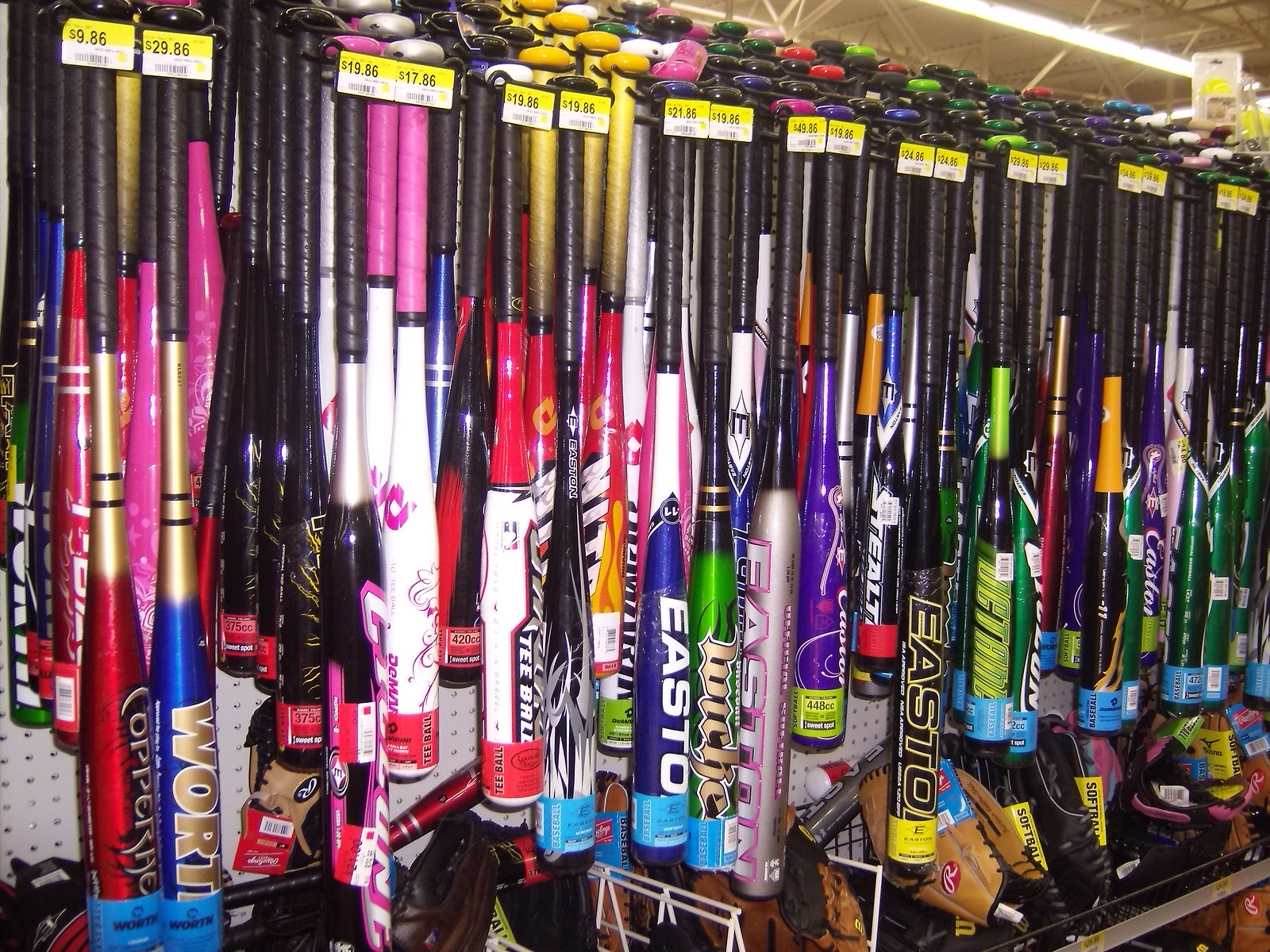The image depicts a section in a sports store, possibly a Walmart, showcasing a large, organized display of baseball and softball bats. The bats are hung vertically, with their handles slotted into metal tines, creating orderly rows sorted by price tags, which range from around $9.86 to $50. The bats come in a plethora of colors, including shades of blue, red, green, white, purple, gold, pink, black, yellow, and orange, with several multicolored options. Many bats are branded Easton, although some branding details are obscured. Below the bats, there are shelves holding various baseball gloves. These gloves, available in colors like black, tan, and pink, are arranged neatly, with some displayed in baskets. The store's industrial ceiling, featuring crisscrossing metal rafters, and a beam of light in the upper right corner, add to the setting's typical retail atmosphere.